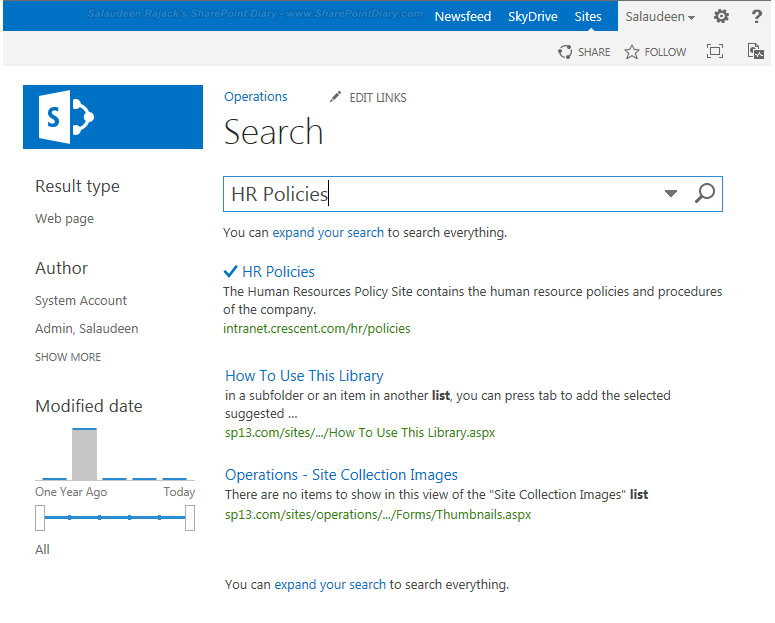The image captures a screenshot from the SkyDrive site interface. At the top, a prominent blue banner displays navigational options including "Newsfeed," "SkyDrive," and "Sites," alongside the logged-in user's name, which is "Saladin." Adjacent to the user's name are icons for settings (cogwheel) and help (question mark). Directly below, a grey sub-banner presents a series of icons on the right for functions like "Share," "Follow," and "Full Screen."

On the left side of the screen, beneath the blue SkyDrive banner, various headings are listed, such as "Result Type," "Webpage," "Author," "System Account," and "Admin." A "Show More" link and a "Modified Date" filter are also visible. To the right, under "Operations," a search dialog box allows users to enter queries.

In this instance, the user has searched for "HR policies," and the search results appear below. The results include multiple documents related to HR policies, such as a specific document from "intranet.crescent.com/HR/policies" about HR policies, a document on how to use the library, and another related to "Operations Site Collection Images."